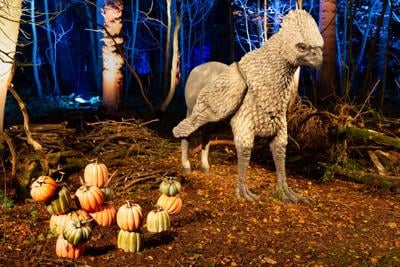The photograph captures an eerie, fantastical scene set in a dark, wooded forest, illuminated by spotlights that cast an eerie blue glow on the surroundings. The central focus of the image is a peculiar, mythical creature resembling a hippogriff. It stands in a small clearing, its body a mix of bird and horse features. The creature has two front legs akin to those of a large bird, with talons, and two hind legs resembling a horse's, complete with hooves. Its gray feathers contrast with its almost ape-like face, which is adorned with large orange eyes and a short beak. The forest background is lit to enhance the spooky atmosphere with dark brown grit, old trees, and scattered twigs. In the bottom left corner, there is a collection of small pumpkins and gourds, in shades of orange and green, stacked oddly. The overall ambiance is haunting, with a mix of natural elements and fantastical, edited details creating an unsettling yet captivating scene.